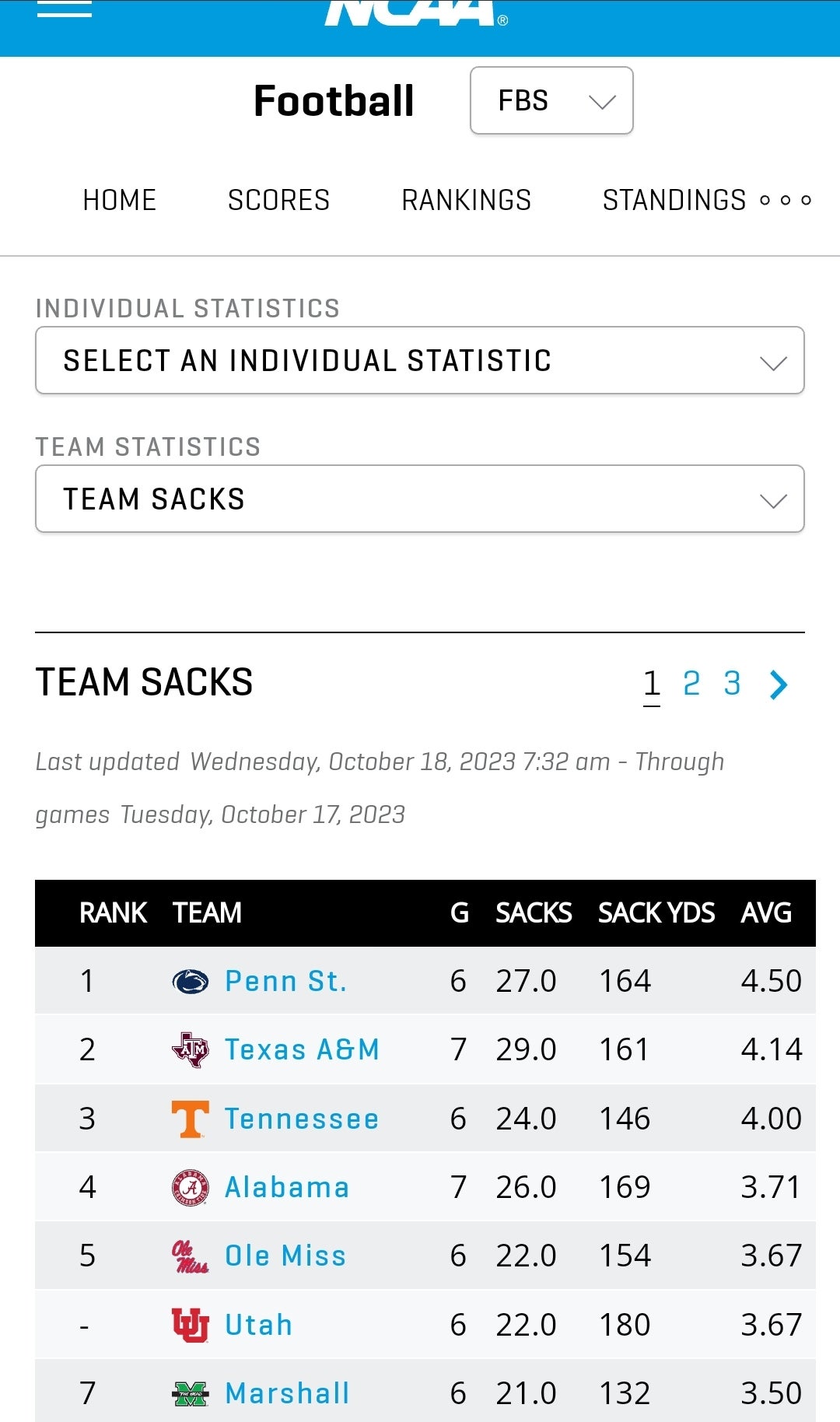The image showcases an application interface, likely related to fantasy football or NCAA football based on the visible elements. At the top of the screen, there's a header labeled "NCAA," accompanied by three vertical dots indicating a menu for additional options. Directly below the header, a large title reads "Football," with a button next to it that appears to allow users to switch leagues, currently displaying "FBS."

The user interface is organized into multiple sections. The first section offers four menu items: "Home," "Scores," "Ranking," and "Standings." Below this is another segmented control with two options: "Individual Statistics" and "Team Statistics," each represented by separate tabs that users can switch between.

Further down, a bordered section labeled "Team Sacks" presents another set of options where users can scroll through different pages. This section displays detailed information about each team's performance, including their ranking, number of sacks, sack yards, and average statistics for what appears to be the current week or game period.